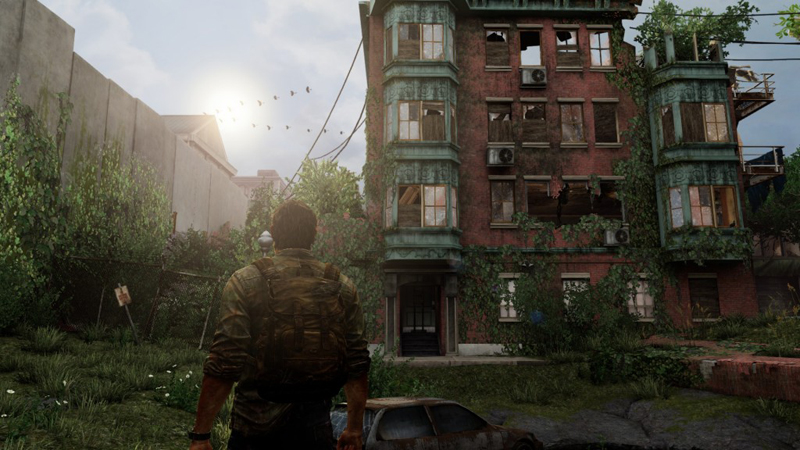In this outdoor scene, a cloudy sky with glimpses of sunlight breaking through serves as the backdrop. The ground is covered in lush greenery and partially enclosed by a chain-link fence, which supports a tilted sign with a white background and red writing. The central focus is a man dressed in army fatigues, including a camouflage shirt and matching backpack, standing with his back to the viewer. He faces a sprawling, dilapidated brick building that once might have functioned as an apartment complex; this structure, standing several stories high, is marked by broken and boarded-up windows. The top portion of the building is particularly derelict, with indications of fire damage and even trees sprouting from it. A car with shattered windows sits in front of the man, adding to the scene's sense of chaos and abandonment. To the left, another degraded concrete building is partially visible, potentially serving as a jail, school, or mall. Finally, high above, a formation of geese fly in a V pattern, signaling a change in seasons amidst the war-torn, yet oddly vibrant landscape.